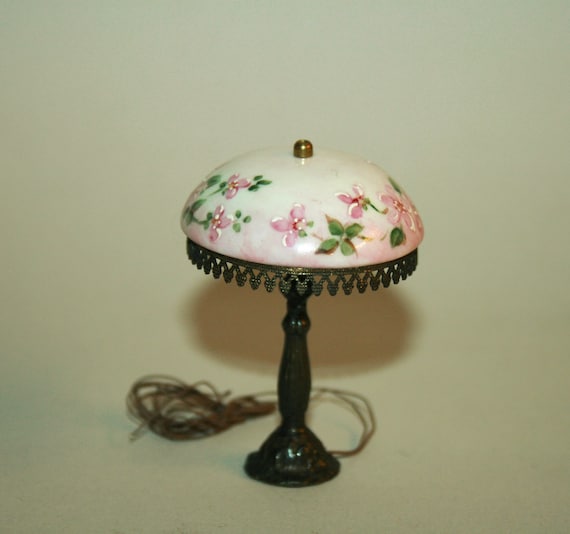This is a photo of an antique Tiffany-style lamp. The lamp features a pedestal base in a dark brown or black color, which may be made from metal or wood. A rolled-up tan electrical cord extends from the bottom of the lamp. The shade, shaped like a dome or mushroom cap, is light-colored and adorned with painted pink flowers and green leaves. A little gold or brass filial tops the shade, adding a touch of elegance. Surrounding the bottom edge of the shade is a dark brown metal filigree design, giving it a scalloped appearance. The background is a pale green or off-white wall, providing a muted contrast to the lamp's intricate details. The overall lighting is slightly dim, enhancing the vintage, antique atmosphere of the scene.